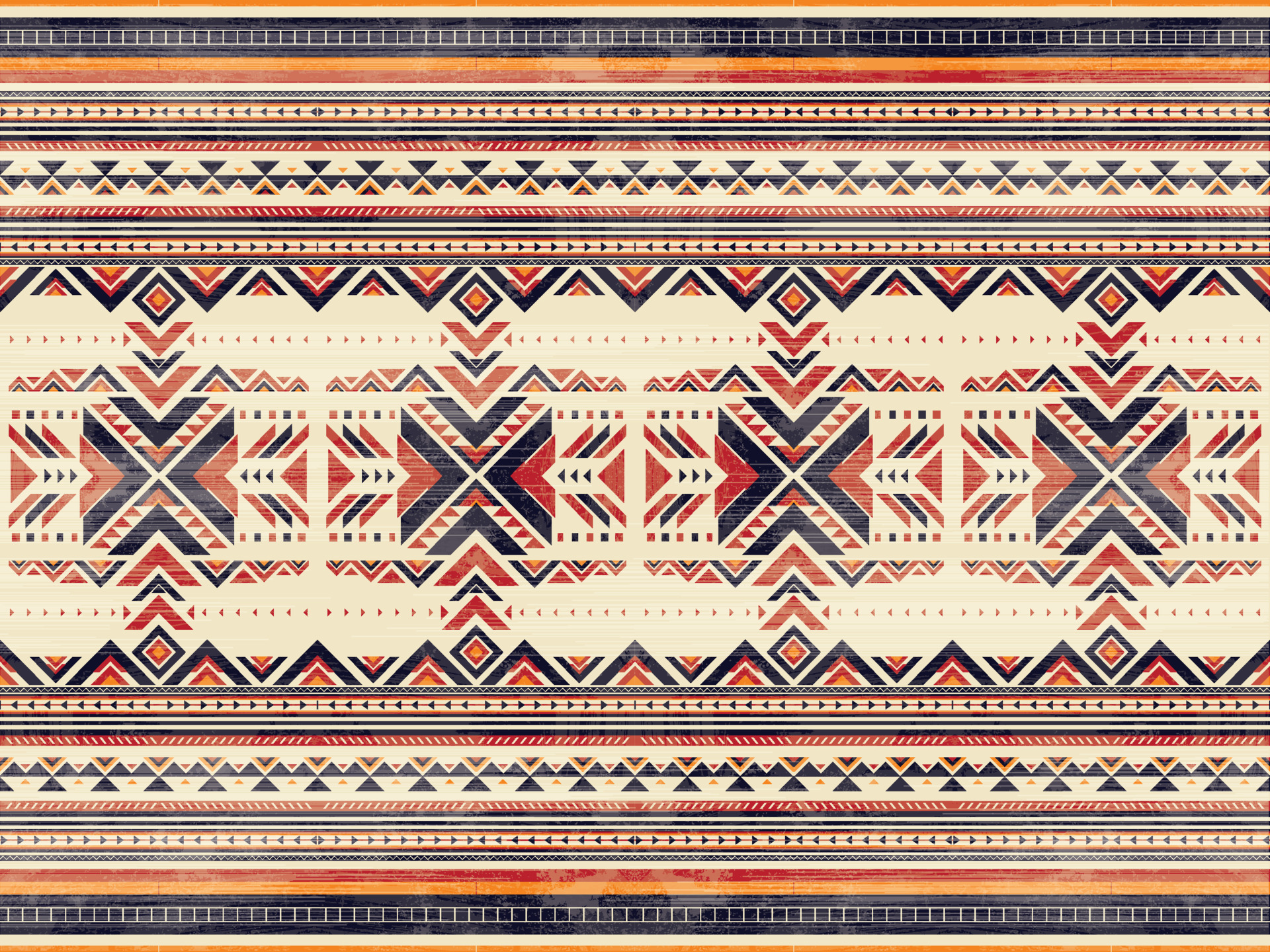The image depicts a detailed, vintage-looking quilt with strong geometric and symmetrical patterns, resembling indigenous or Navajo designs. It primarily features earth tones such as light beige, terracotta, tan, and deep olive green, with additional colors like red, blue, black, yellow, orange, and off-white cream. The central design includes four squares with various X-patterns, where triangles dominate—some being hollow and resembling cottage shapes filled with smaller triangles of different colors. 

The borders are richly decorated, starting with lines of rust tan and off-white cream, followed by black stripes with a silver ladder pattern, and ending with rows of black, red, and yellow triangles. 
A burnt red stripe and layers of arrows and diamond-like textures add complexity to the design. The patterns grow more abstract and larger towards the center, giving an Aztec-like appearance. This tapestry-like piece could be mistaken for a woven rug and features a highly symmetrical layout, making it versatile for various decorative uses.